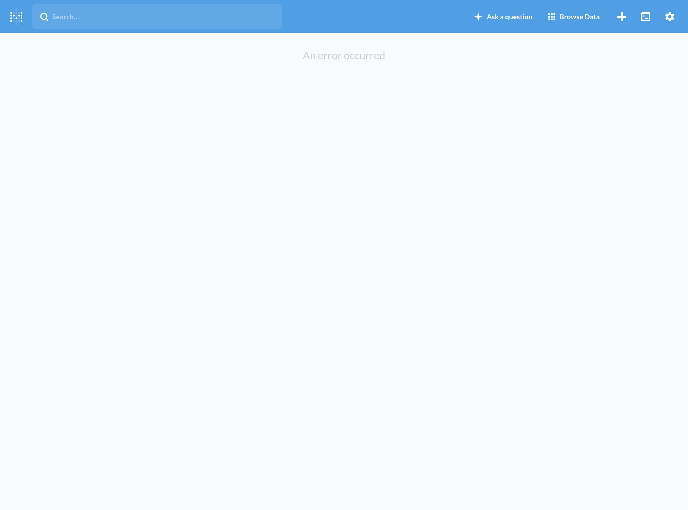The image features a clean white square interface with a distinctive blue border at the top. The top section prominently displays the letter "M" followed by a search bar, complete with a search icon. Next to the search bar, there is functionality to add a request labeled "Requiem Bronson Delta," along with icons for a calendar and settings. Towards the bottom of the square, a message in clear text indicates that "An error has occurred."